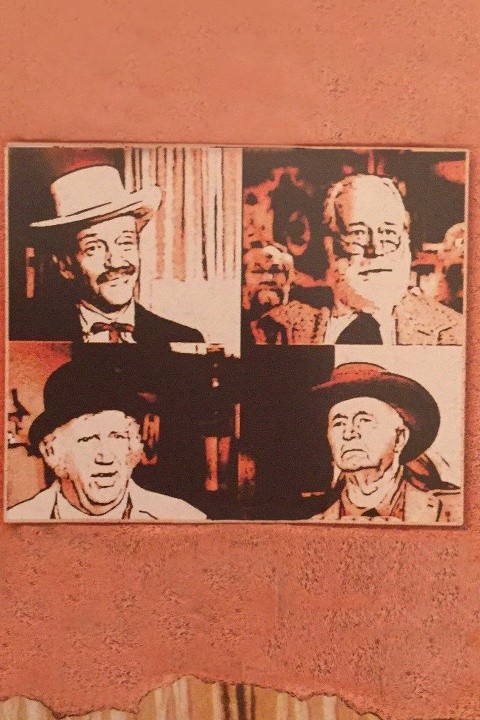This image is a collage of four black-and-white photographs arranged in a 2x2 square. Each photograph depicts a different white-skinned man, possibly actors in an old-time movie, with a reddish-pink hue giving a vintage feel to the entire composition. The collage is glued onto an old, salmon-colored paper that has a torn bottom edge, revealing dark and light wood paneling underneath.

- **Top Left:** A mid-aged man with a mustache, wearing a white hat, a black jacket, and a little black bow tie. He faces slightly to the right.
- **Top Right:** An elderly man with receding white or gray hair, glasses low on his nose, a full mustache, and a beard. He wears a gray suit and black tie.
- **Bottom Left:** Another gray-haired elderly man, donning a black derby hat. He is facing towards the right and appears to be wearing all white.
- **Bottom Right:** An old man with a black cowboy hat, clean-shaven and slightly bald, gazes to the left with his head tilted up slightly. He wears a dressy outfit with a white undershirt and a tie.

Each photograph has distinct backgrounds with shades ranging from black to red, adding to the contrast and vintage collage-inspired aesthetic.